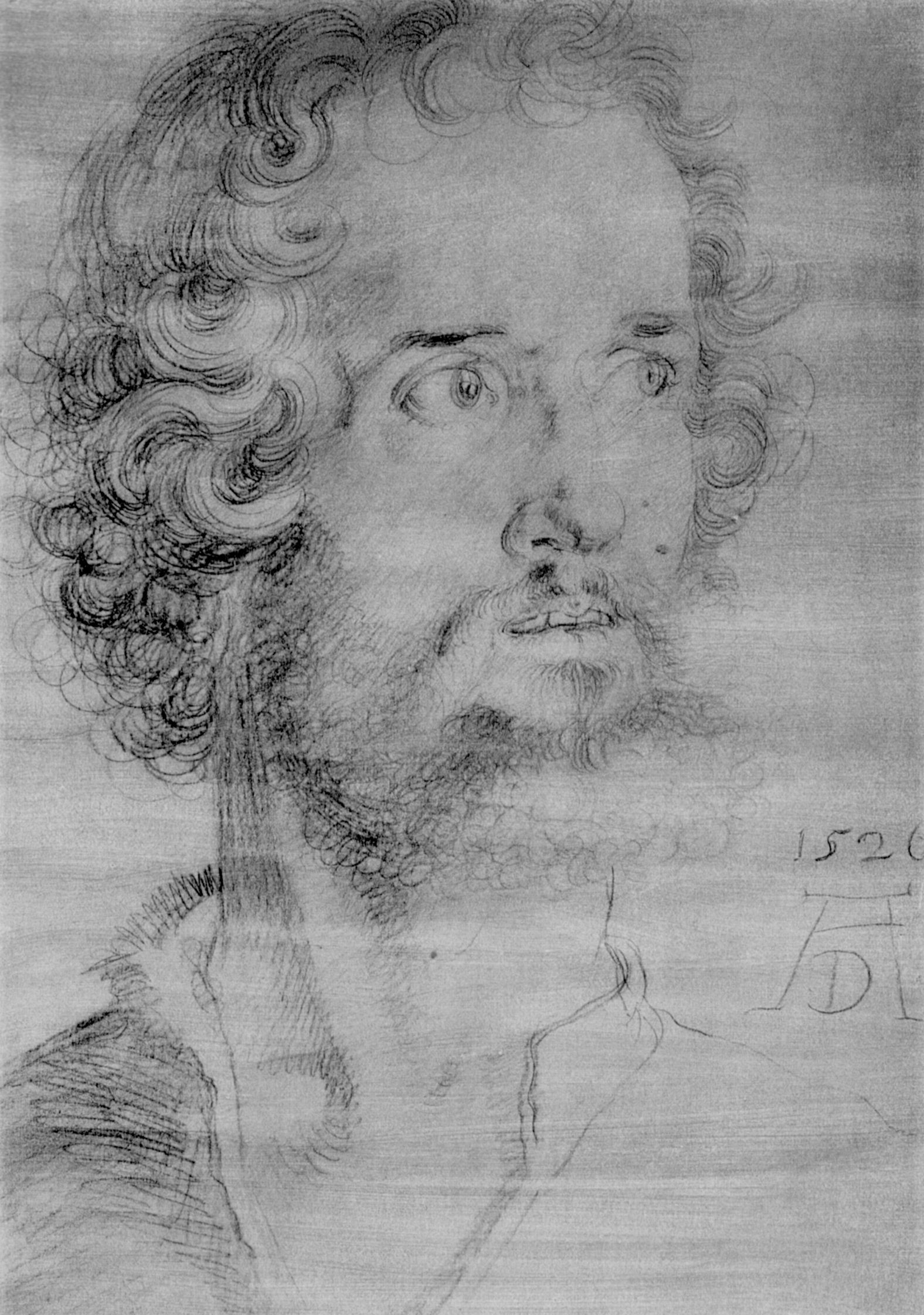This black and white pencil drawing, dated 1520, features a close-up of a man's face, turned slightly to his left. Notable for its historical style, the portrait shows a man with wide, light eyes that display a mix of concern and contemplation. His curly hair falls below his ears, and he sports a wiry, curly beard along with a thin mustache. His lips are slightly parted, revealing his teeth, and his mouth appears to be hesitant or pursed. The man wears a white shirt, visible just below his neck, and the drawing includes the numbers "1520" along with a signature resembling an "A" over a "D." The image suggests a reference drawing, possibly intended for later elaboration, capturing a moment of trepidation or wary alertness on the man's expressive face.